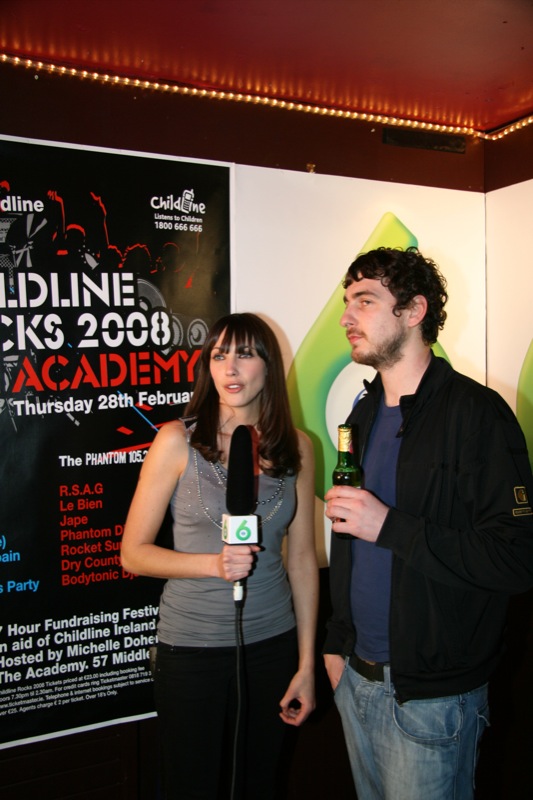In the image, a woman and a man stand together, appearing to be in a press setting at a movie theater. The woman, who seems to be a reporter, is holding a tall microphone with a white base marked with the number 6, likely indicating the channel. She has chest-length black hair with bangs and is dressed in a gray sleeveless top and black pants. The man next to her, donning a black jacket over a blue t-shirt with blue jeans, has short curly hair, a light beard, and is holding a green beer bottle, suggesting he might be interviewed by the woman. 

They are positioned in front of a partially visible poster that contains several pieces of text. The text on the poster includes phrases such as "Thursday, February 28th," "Academy," "fundraising festival," "ChildLine," and "2008." It seems that the event they are attending relates to a fundraising activity for ChildLine, possibly titled "The Anthem." Additional visible details include the event taking place at "The Academy" and being hosted by Michelle. The décor around them includes green structures, a stream of lights, and a red ceiling.